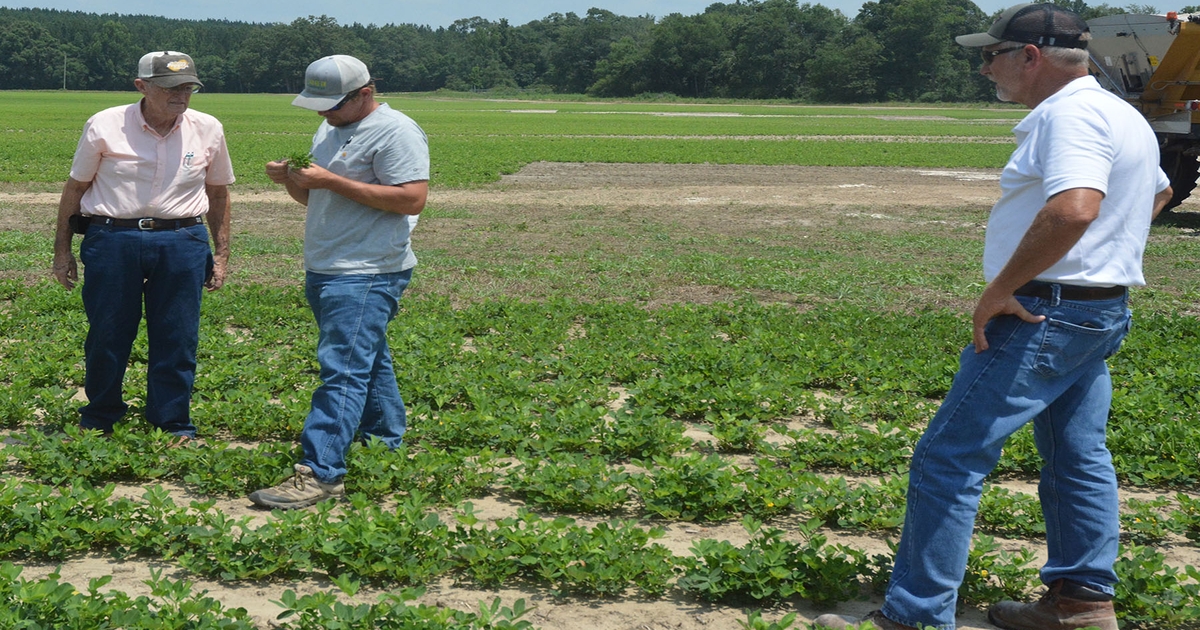In this photograph, three farmers are standing in a large, green farming field under a clear sky. They are all dressed in blue jeans, work boots, and baseball caps, reflecting their hard-working lifestyle. Two of the men appear to be much older, likely in their 60s or 70s, while the third man in the middle looks to be in his 30s. 

The older gentleman on the far left is wearing a light beige button-up shirt and eyeglasses, intently examining what the man beside him is holding. This younger man in the center, wearing a gray or white shirt, has pulled some greenery—possibly a crop sample—out of the ground and is discussing it with the others. The man on the far right, sporting a white shirt and sunglasses, stands with his hand on his hip, observing the scene. 

Behind them, a tree line stretches across the background, encapsulating the spacious farming area. To the far right of the image, just barely visible, there is a yellow tractor with a white container, indicative of the farm's operations. From their clothing to their stance, their demeanor suggests they are investigating the health of the budding crops, possibly looking for signs of insect infestation or drought. The mixture of old and young among these farmers showcases the blend of experience and vigor in agriculture.